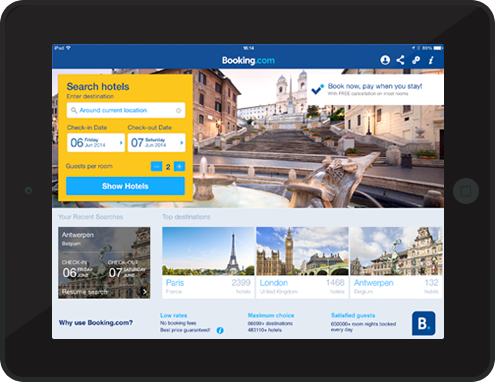A high-resolution image of a black tablet, oriented horizontally, captures the user interface of bookie.com. The screen showcases the website's search functionality, prominently featuring a large yellow "Search Hotels" button. Surrounding this area are date selection buttons and a text field for entering location names. To the right, an image of a picturesque place with stone steps adds a visual appeal.

Beneath the search bar, a section highlights popular destinations, with buttons displaying iconic names such as Paris, featuring the Eiffel Tower, and London, with the distinctive Bell Tower. Other top destinations, including Antwerpen, are also listed in smaller text.

Lower on the screen, various interactive buttons offer users the ability to explore different categories and frequently asked questions about bookie.com. The website's interface includes additional utility buttons at the top right, such as profile, options, share, settings, and information icons.

The top of the tablet screen shows essential device information, like the current time and battery status, ensuring a complete and functional browsing experience.